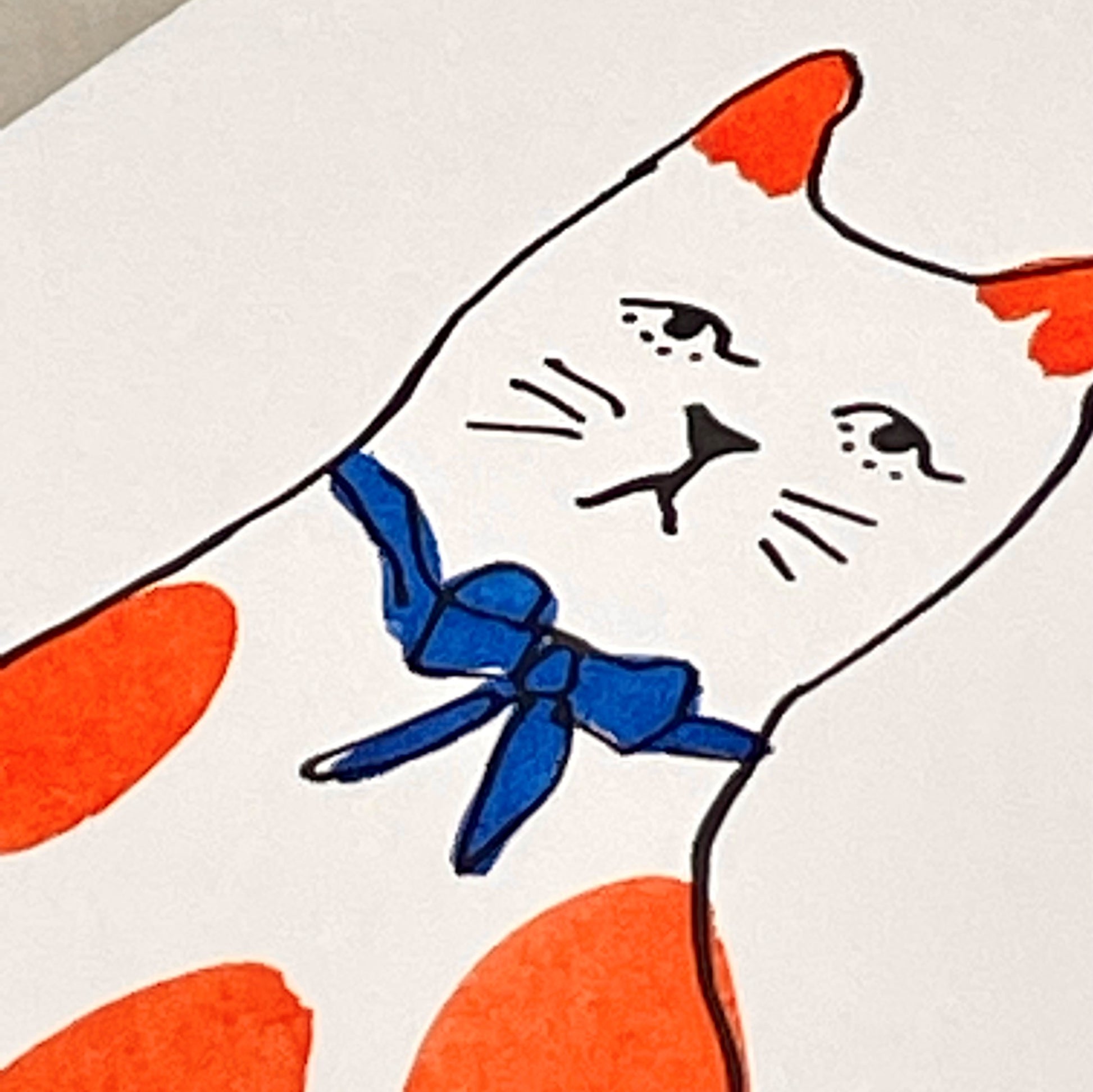The image captures a hand-drawn marker illustration of a cat, positioned on a light gray, likely table or desk surface, visible in the top left corner of the frame. The photograph is taken from a slightly angled top-down perspective, causing the top of the cat to point towards the top right and the bottom towards the bottom left. However, the framing cuts off part of both the cat and the paper, suggesting the image's focus is primarily on the cat's upper body.

This illustration features a predominantly white cat adorned with orange-tipped ears and several orange spots: one on each shoulder and one on the chest. Around its neck is a blue ribbon tied into a neat bowtie. The cat's facial details include black eyes, each with a couple of hand-drawn dots beneath, a small triangle-shaped nose followed by an inverted V-shape mouth, and three whiskers on each side of its face. The use of marker is evident in the coloring, showing bleeding edges where the ink has spread over the white paper.